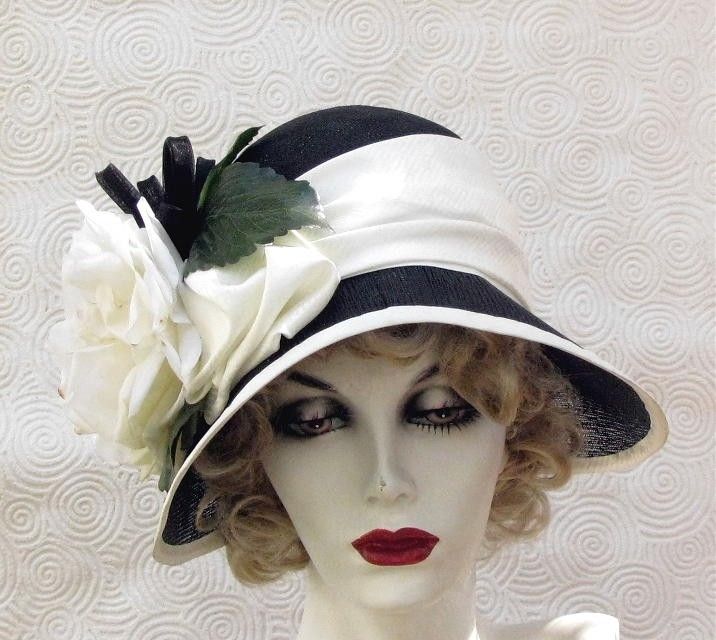This photograph features a mannequin head with detailed makeup and accessories. The mannequin has a white face with prominent dark gray eye shadow and bright red lipstick, giving it an old-style appearance. A short curly blonde wig adorns its head, beneath a chic hat that alternates between black and white: black at the top, white in the middle, and black again around the rim. The mannequin's green eyes are directed downward, adding a contemplative vibe to its gaze. To the left of the mannequin is a large, white artificial flower with green leaves extending from it. The background is a swirled pattern of overlapping circular designs etched into a white fabric, which adds an intricate and elegant backdrop to the scene. This setting evokes a blend of vintage glamour and modern artistry.